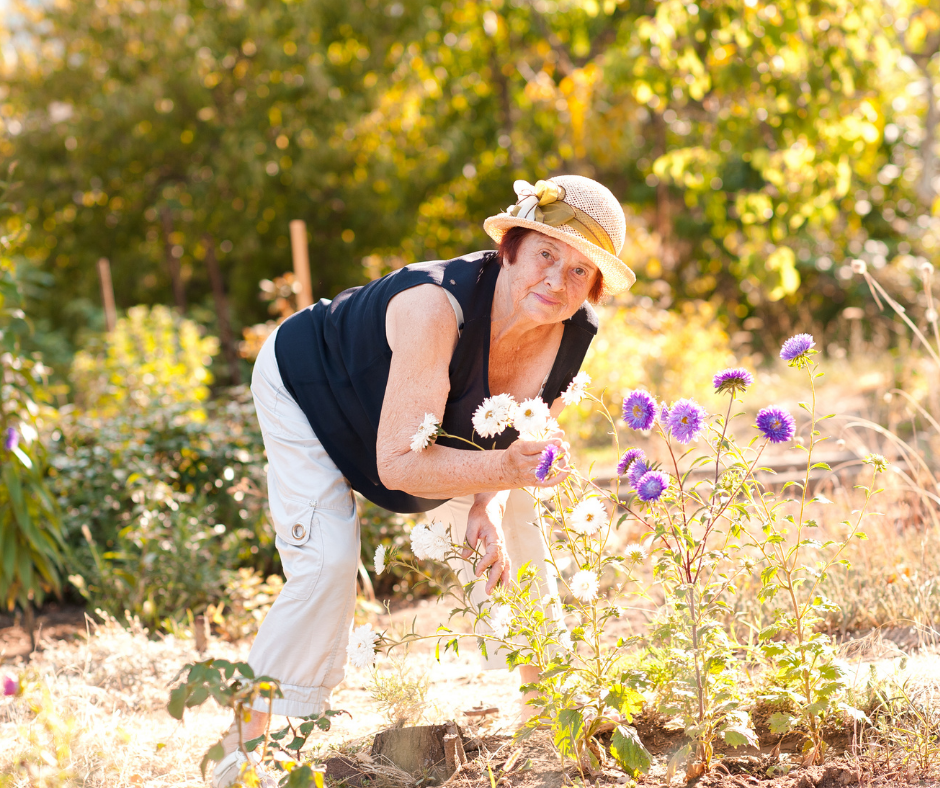In this photo, we see an older woman, around 70 years old, bent over in a garden, carefully picking flowers. She is dressed in a blue sleeveless shirt and white cargo pants with stretchy cuffs, and she wears a small-brimmed straw hat adorned with a yellow ribbon and a white bow. The woman holds freshly picked daisies in her hands and is surrounded by vibrant purple and white flowers, their green leaves and brown stalks adding rich texture to the scene. The background is a lush, tree-lined area with thick, full trees partially obscured by a soft focus. The sun shines through the foliage on the right side of the image, illuminating the scene. Wooden poles, likely used for supporting plant vines, are visible among the overgrown greenery, contributing to the expansive, almost boundless feel of the garden.